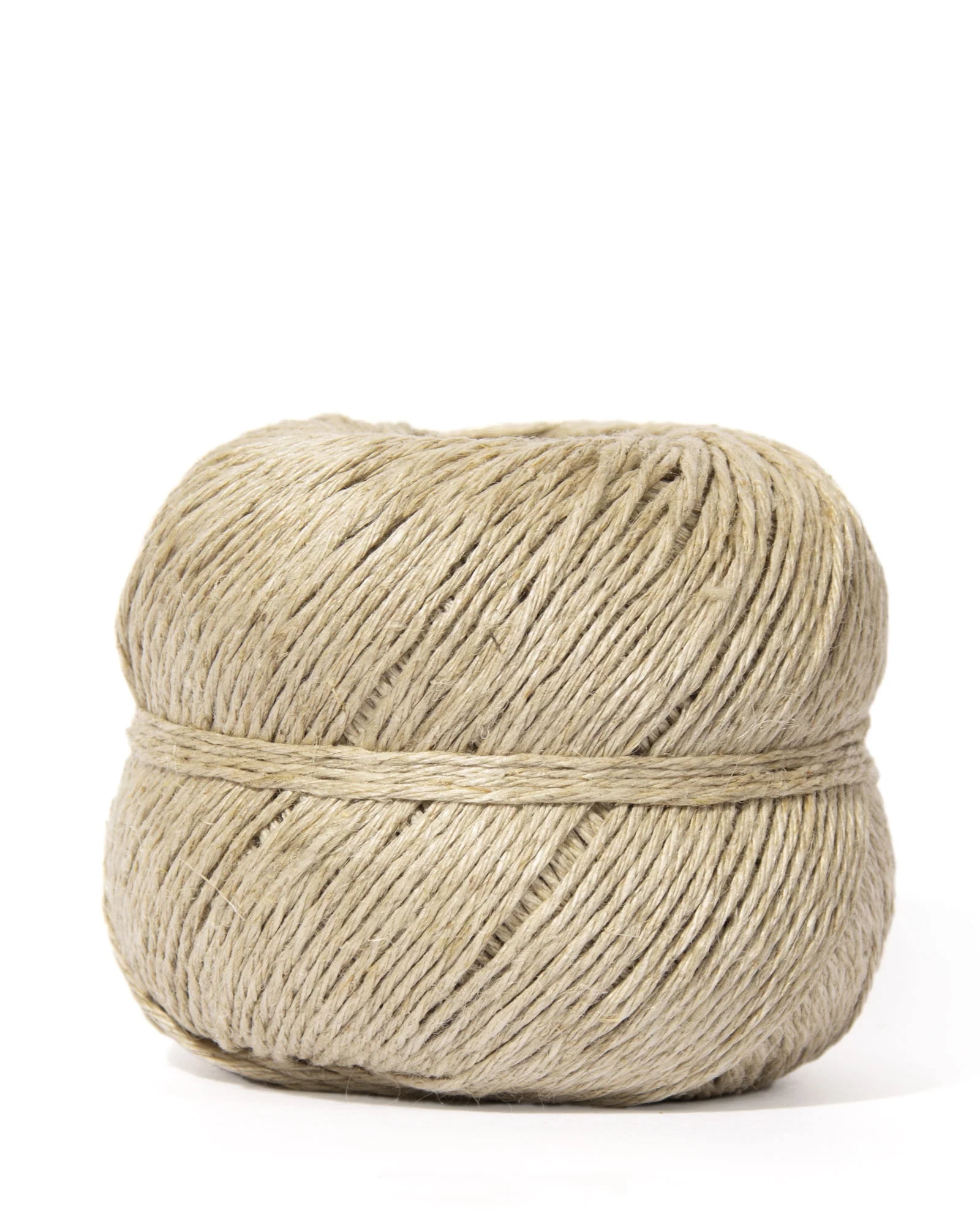This is a highly detailed vertical image depicting a new, tightly wrapped ball of twine. The ball of twine, essentially cylindrical but slightly wider than it is tall, rests on a pristine white background with a faint shadow visible on the lower right side. The twine appears beige and has a rough texture, akin to the kind one might use for packaging. The twine is meticulously wrapped in diagonal lines, almost perfect but with slight spaces in between, creating a visually striking pattern. Noteworthy are the four tightly pulled strands around the middle, causing the center to cave in slightly while the top and bottom bulge outward. The entire composition is simple, focusing solely on the ball of twine without any extraneous elements, highlighting its new, unused condition.